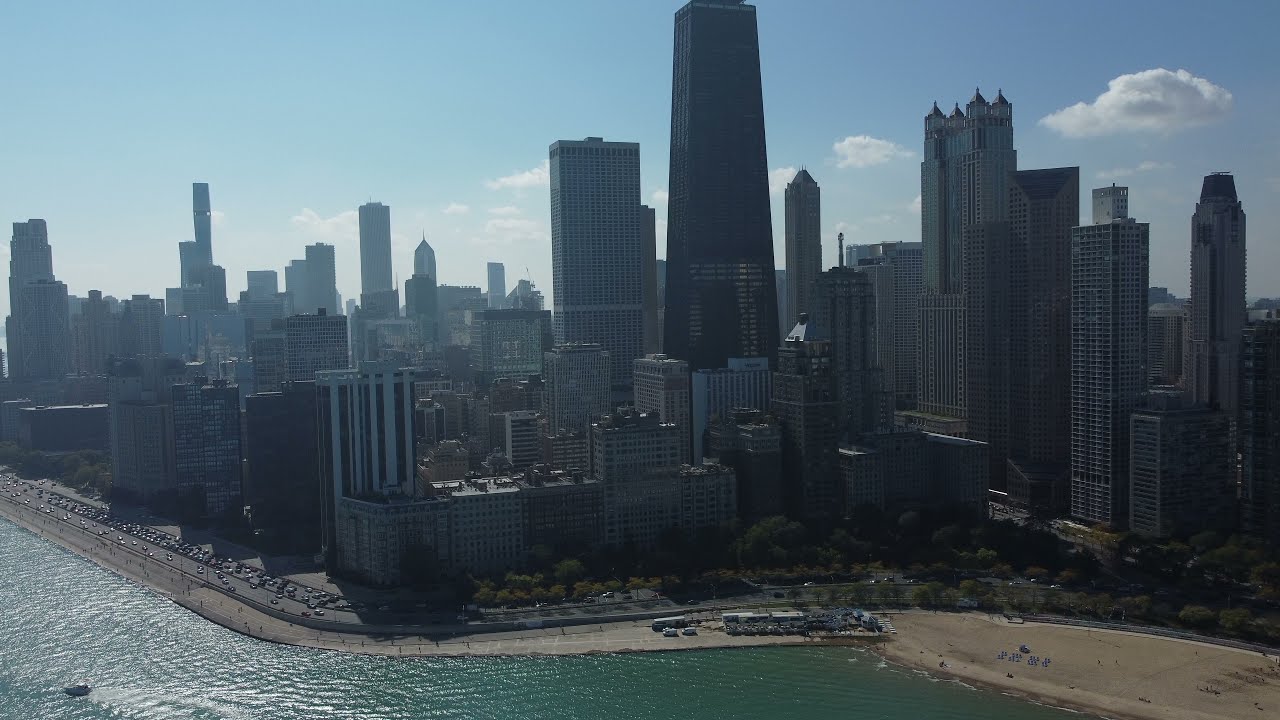This photograph captures the stunning skyline of Chicago as seen from Lake Michigan. Dominating the scene are numerous tall skyscrapers, including the iconic John Hancock building, some with triangular tops and others with flat ones. The buildings, many silhouetted against the sunlit sky, stretch almost to the water's edge. A long road with two-way traffic runs along the narrow strip of land separating the skyscrapers from the lake. On the right side of the image, there's a broad sandy beach leading into the deep turquoise waters of Lake Michigan, where a small white boat sails near the bottom left corner. A variety of vehicles, including cars and larger ones like buses, are scattered along this strip, with some parked on the side near the water. Sparse white clouds dot the mostly blue sky, completing this captivating urban and waterfront scenery.